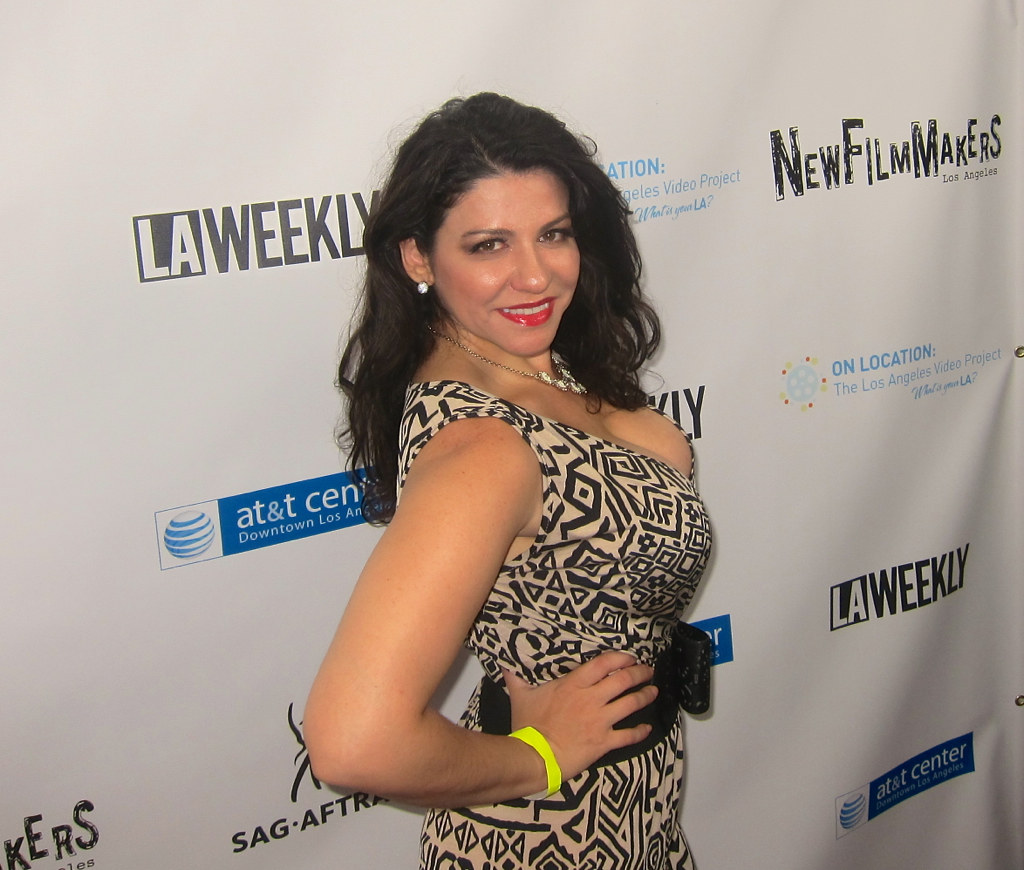The photo captures a Caucasian woman with long, flowing black hair posing confidently at what appears to be a red carpet event. She is dressed in a striking black and cream dress adorned with various geometric patterns, including diamonds, squares, and arrows. The dress is cinched at the waist by a wide black belt, partially hidden by her hand, which rests on her hip. Her other arm, adorned with a light yellow armband, hangs by her side. She accessorizes with a jewel necklace partially obscured by her hair, a pearl earring, and wears bold red lipstick and eye makeup, giving her a glamorous look as she looks directly at the camera. The background features a white backdrop with an array of logos, such as LA Weekly, AT&T Center, New Filmmakers, SAG-AFTRA, Downtown Los Angeles, On Location, and the Los Angeles Video Project, indicating that she is likely attending a high-profile event or award ceremony.